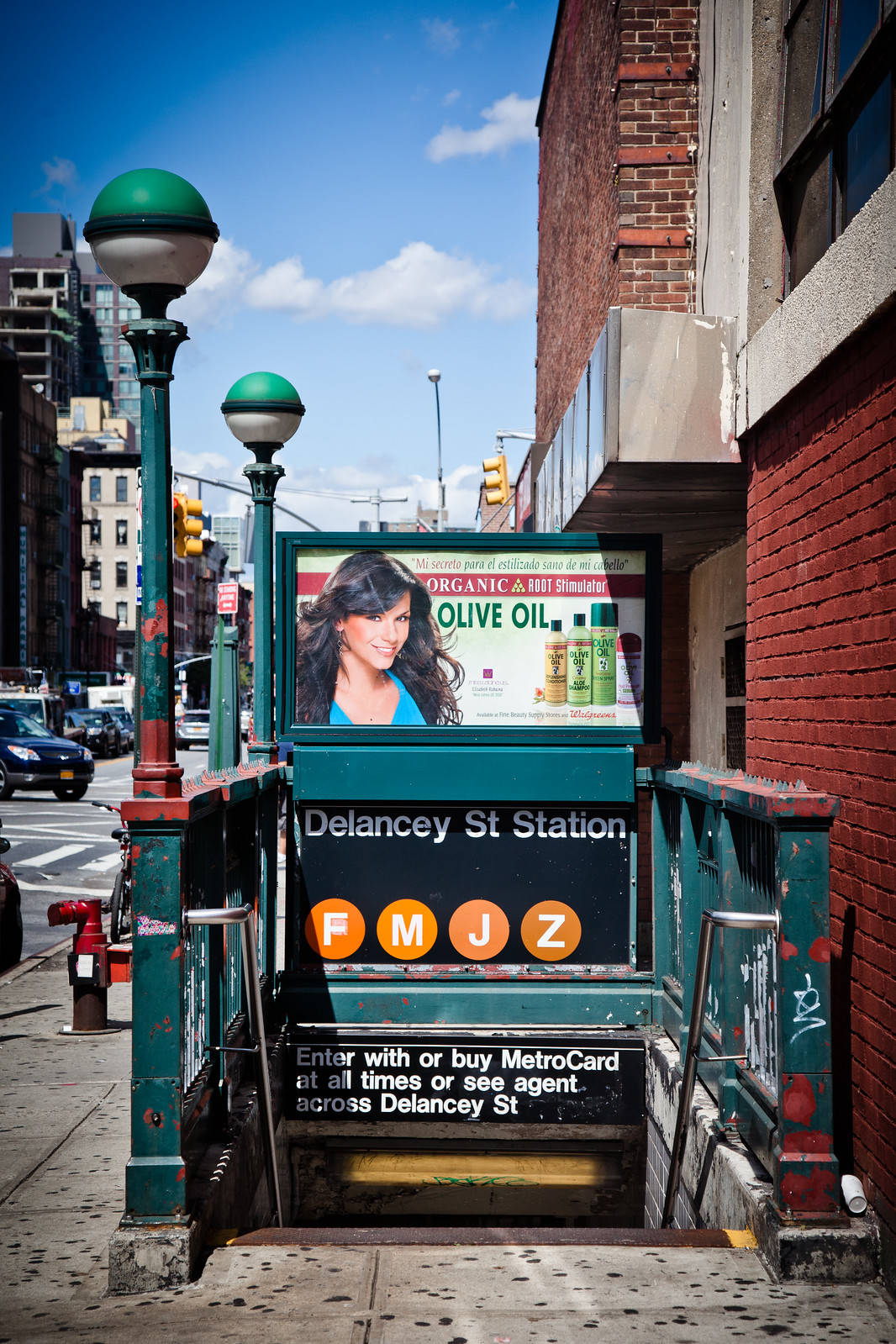This vibrant photograph captures a typical bustling scene at the entrance of Delancey Street Station in New York City. The foreground is dominated by the entrance to the subway station, where stairs descend into the urban underground. The stair rails, painted in a mix of green and red and adorned with graffiti, frame the scene, leading the eye downward. Two light posts, featuring globe-shaped lights in green and white, mark the entrance.

Above the entrance, an advertisement for an organic root stimulator olive oil featuring an attractive woman with product bottles to her right takes center stage. Directly below this ad, the Delancey Street Station sign is prominently displayed, accompanied by the subway lines F, M, J, and Z, each encircled in their respective orange circles. The sign informs passengers that they must enter with a MetroCard or visit the agent across the street, underscoring the self-service nature of this station. 

The backdrop is a lively urban tapestry with moderate-height brick buildings in hues of red, interspersed with railings and various signs in white, orange, black, and green. The street to the left is dotted with moving cars, indicating the never-ending flow of city life. In the top left corner, more buildings line the opposite side of the street, while the sky, a light blue with scattered white clouds, suggests it is daytime. This detailed and richly colored scene epitomizes the dynamic and busy atmosphere of a major city's subway entrance.